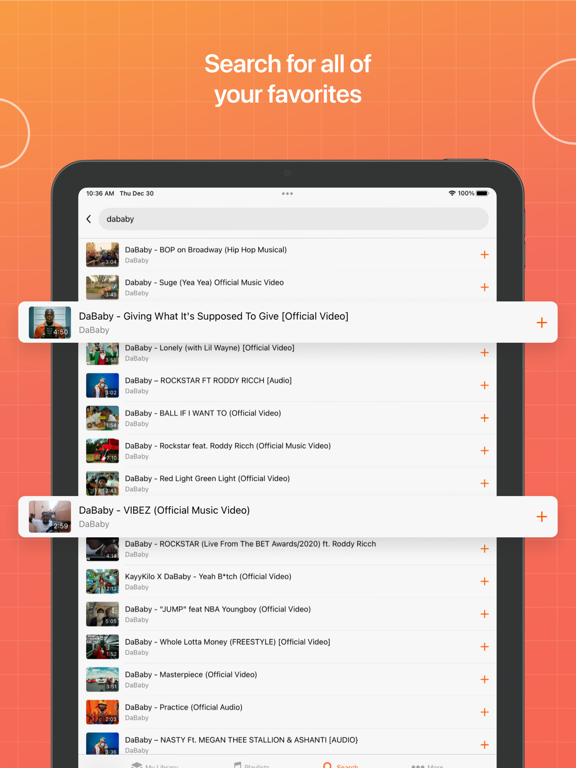The image features an iPad against a vibrant orange background. The screen of the iPad displays a search interface with the caption, "Search for all of your favorites." The display shows several notable music titles from DABABY, including "BOP on Broadway," "Hip Hop Musical," "Shuggie," "Yeah Yeah," "Offshore Music Video," "Giving What It's Supposed To Give Offshore Video," "Lonely With Lil Wayne Offshore Video," "Rockstar Featuring Roddy Ricch," "Vibes Offshore Music Video," "Rockstar Live from the BET Awards 2020 Featuring Roddy Ricch," and "Jump Featuring NBA Youngboy Offshore." 

In the top left corner of the screen, the device shows the current time as 10:36 AM and the date as Thursday, December 30. The top right corner indicates a full battery with a 100% charge and a strong Wi-Fi connection icon.